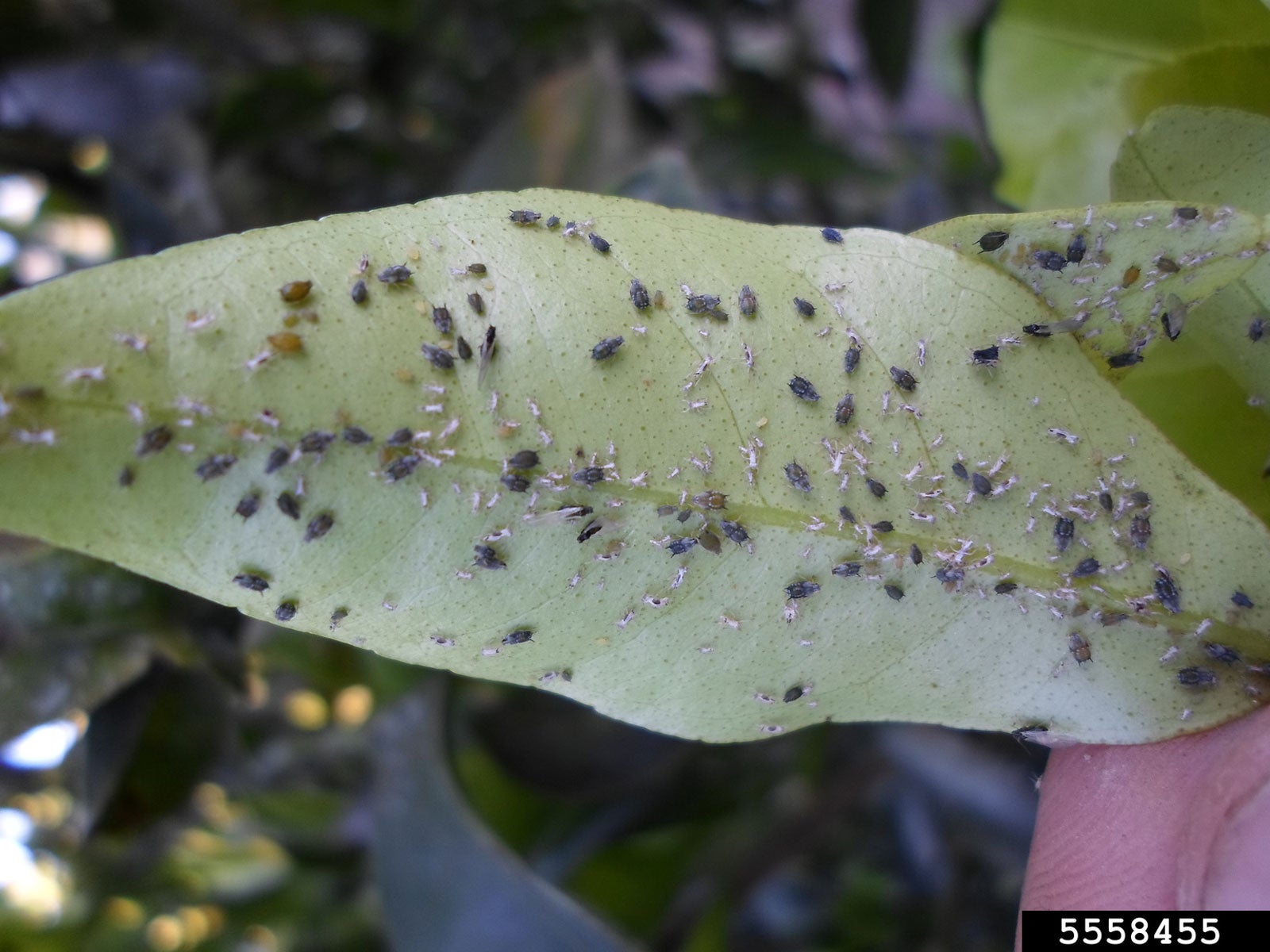The image depicts a detailed, close-up view of a green leaf that appears to be held up by the tip of someone's finger, visible in the bottom right-hand corner along with a black rectangle containing white lettering that reads "555A455." This central leaf, which is surrounded by a blurred, forest-floor background, hosts an array of tiny insects. Predominantly, there are small, white, ant-like insects, and darker bugs, reminiscent of fleas or fly larvae, scattered across the leaf's surface. The insects, varying in size and color, appear to be either hatching or feeding on the leaf. Despite their different appearances, they seem to coexist on this light green foliage, suggesting a complex, interconnected ecosystem.